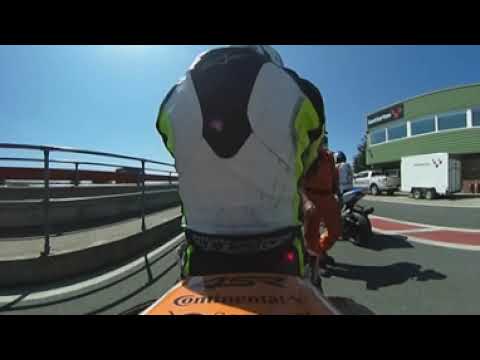This detailed outdoor photograph, taken from a slightly distorted, bubble lens perspective, captures a dynamic motorcycle scene on a paved roadway. Centered prominently, a person in a black, white, and green jumpsuit and a matching white, black, and blue helmet stands holding the handlebars of a motorcycle, which features bright orange text reading "45 Continental." In front of this rider is a man in a blue short-sleeved shirt, facing the camera. Surrounding them are several other motorcycle riders, three of whom are visible in the background, racing towards the right side of the image. The road features a yellow line on the right and a white stripe running from left to right. The scene is framed by a solid black border at the top and bottom, and the sky above is clear, indicating a bright, sunny day with minimal clouds.